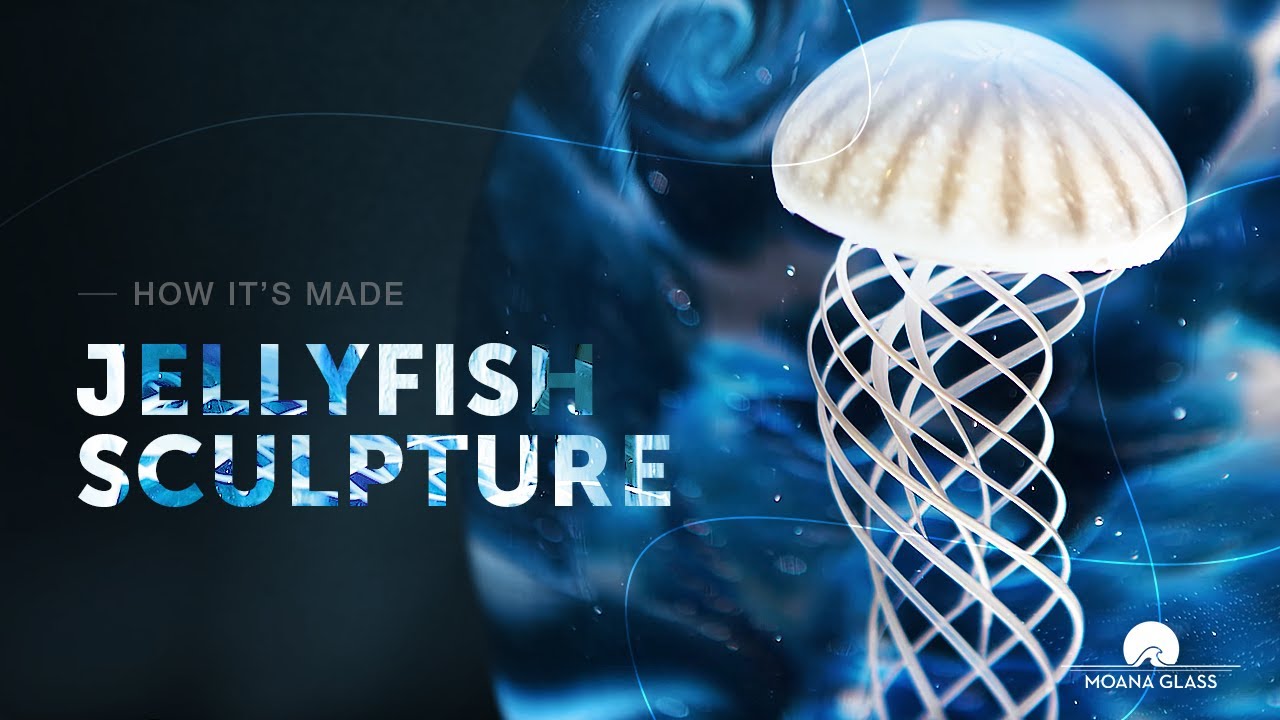This is a detailed color advertisement for Moana Glass, featuring a glass jellyfish sculpture. The central focus is a luminous, white jellyfish with tentacles that twist in a pattern reminiscent of DNA. These tentacles form a tight spiral inside a cylinder, suggesting movement. The background is a mesmerizing blend of bluish-white swirly and watercolor patterns. On the left side of the image, bold, gray text reads "How It's Made," followed by "Jellyfish Sculpture" in block letters. These letters feature a gradient array from white to bluish-white to green, with intricate sea creature scenes nested within. In the bottom right corner, a logo with a wave design accompanies white text that reads "Moana Glass."